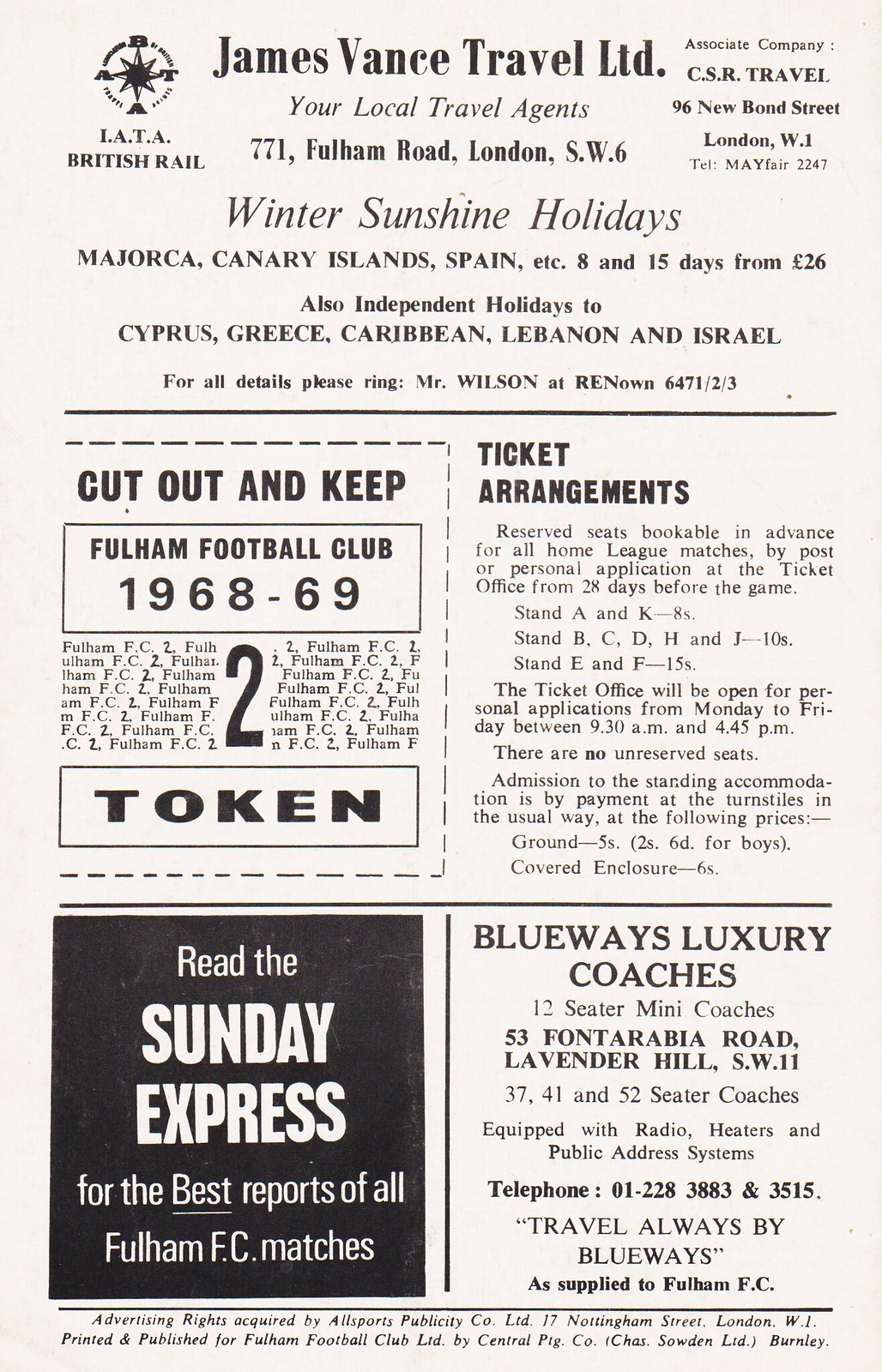This image depicts a detailed page full of advertisements, divided into three main sections. At the top, the first section showcases an ad for James Vance Travel, LTD, described as "Your local travel agents" located at 771 Fulham Road, London, SW6. This ad also includes additional details such as the associate company CSR Travel located at 96 New Bond Street, London W1, offering winter sunshine holidays to destinations like Majorca, the Canary Islands, and Spain, with varying lengths from 8 to 15 days and prices starting at 26 pounds. Contact details for Mr. Wilson at Renown 6471-2-3 are provided for further arrangements.

In the second section, the page highlights the Fulham Football Club's 1968-69 season with a bold heading that reads "Cut and Keep Out, Fulham Football Club, 1968-69, Two Token." Below this heading, ticket arrangements are meticulously detailed, explaining that reserved seats for all home league matches can be booked in advance by post or in person at the ticket office starting 28 days before the game. Specific seating sections and prices are outlined: Stand A and K-8, Stand B, C, D, H, and J for 10s, and Stand E and F for 15s. Personal applications for tickets are accepted at the office from Monday to Friday between 9:30 a.m. and 4:45 p.m., with specified prices for the ground and covered enclosures. Alongside this, an advertisement for reading the Sunday Express for extensive Fulham FC match reports is present in white text on a black background. 

The third section on the right side of the page advertises Blue Ways Luxury Coaches. This ad elaborates on the services provided, featuring 12-seater mini-coaches up to 52-seater coaches, all equipped with radios, heaters, and public address systems. The company is located at 53 Fonterra Arabia Road, Lavender Hill, SW11, and emphasizes its connection to Fulham FC. Contact information includes telephone numbers 01-228-3883 and 3515. Lastly, there are credits indicating that advertising rights belong to All Sports Publicity Co, LTD, based on Nottingham Street, London, and that the printing was done by Central PTG Company.